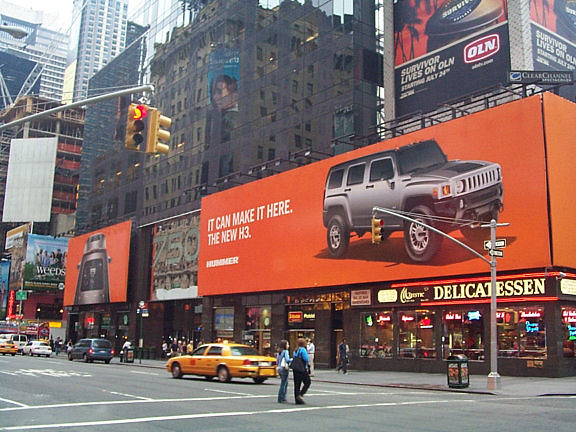This image captures a bustling intersection in a vibrant metropolitan area, likely New York City, reminiscent of a scene from Times Square. Dominating the foreground are two individuals crossing the street at a crosswalk beneath traffic lights, which are currently showing red. Close to them is a taxi cab, with a few other cars, including a blue minivan, dispersed along the multiple lanes of the road running to the left. The street is flanked by a series of towering buildings on the right, their base floors adorned with a variety of storefronts, restaurants, and delis, including one prominently labeled 'Delicatessen.' Above this delicatessen, a giant electronic billboard advertises the new H3 Hummer with a slogan, "It can make it here," featuring a silver Hummer truck. The tops of the buildings are lined with large, reflective windows, while the scene is alive with a mix of pedestrians and vehicles.